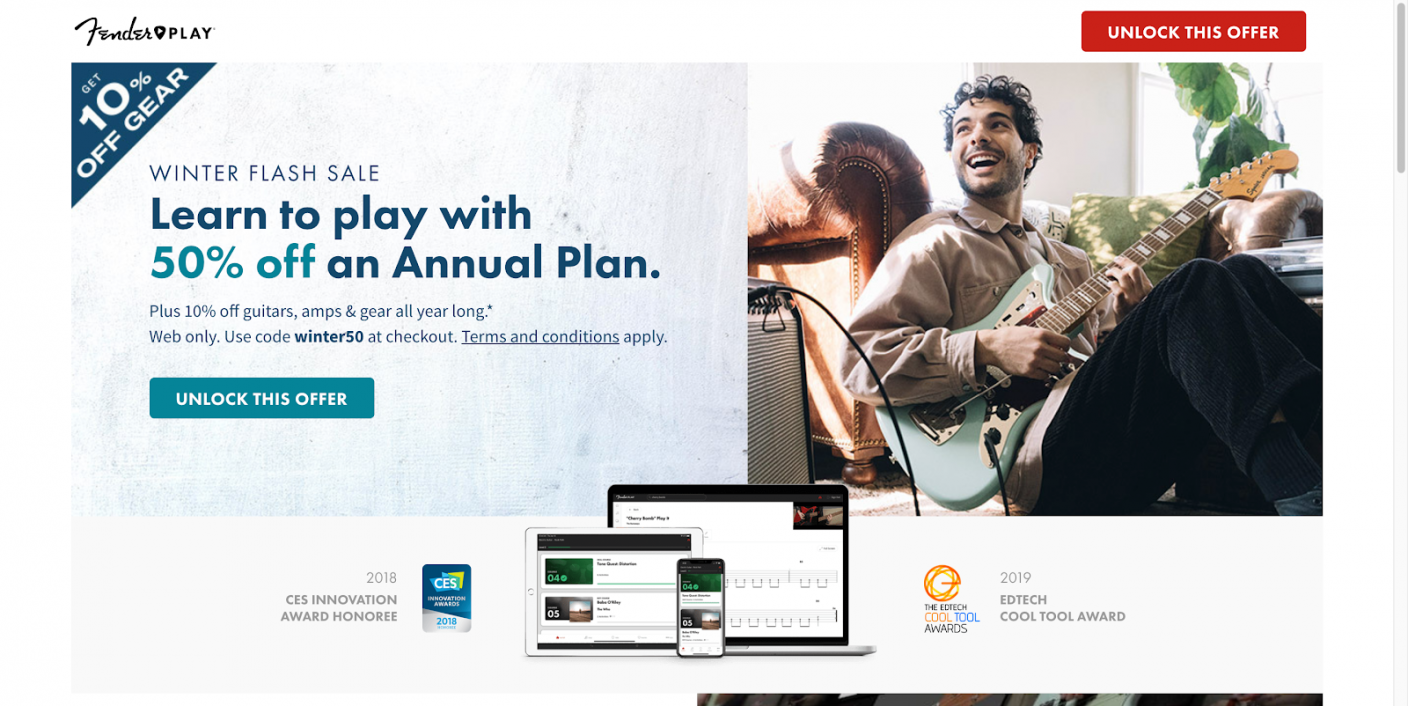**Caption:**

This horizontally oriented image appears as a promotional banner that could be sent via email or viewed on a web page on both computer and smartphone devices. The background features a whitish-blue streaked design. In the top-left corner, the text "Fender Play" is visible. Below, a dark teal triangle with white text offers "Get 10% off gear".

Prominently displayed in bold text is the announcement "Winter Flash Sale" and the enticing offer "Learn to play with 50% off an annual plan". In a smaller and less bold font, there's an additional offer: "Plus 10% off guitars, amps, and gear all year long. Web only. Use code WINTER50 at checkout. Terms and conditions apply."

Two prominent buttons labeled "Unlock this offer," one in teal and another in orange, are positioned at the bottom and top-right of the image, respectively.

At the center of the visual, a man with curly black hair, a mustache, and a beard, dressed in a long tan shirt and black pants, is shown playing a guitar while laughing and looking up at someone. Near the bottom, there is an icon of the "CES Innovation Award Honoree 2018", alongside various tablet and iPhone symbols, and another icon indicating the "EdTech Cool Tool Award 2019".